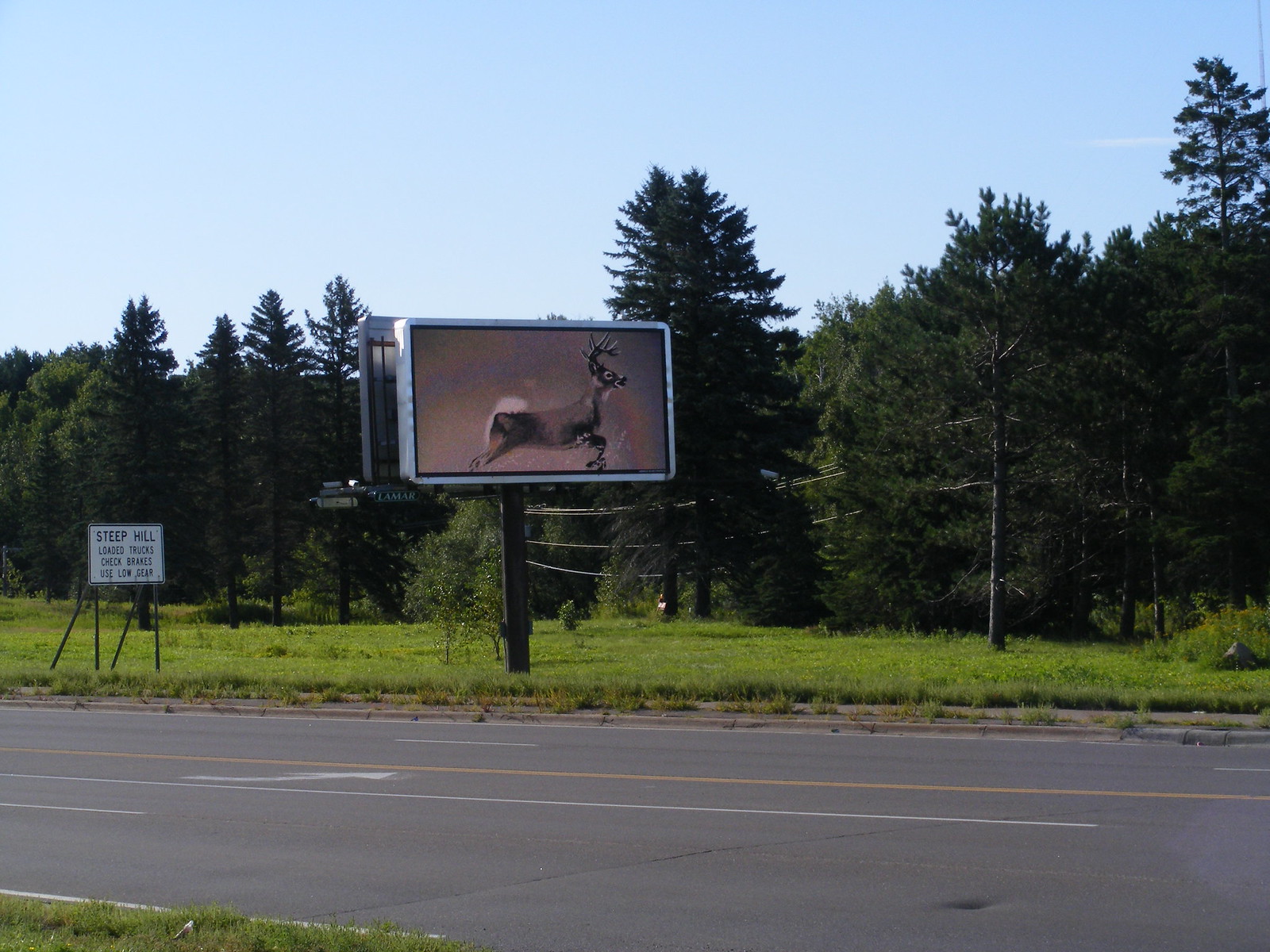The image depicts the side of a forested road with several power lines and a prominent billboard. The white sign reads, "Steep Hill: Loaded Trucks Check Brakes. Use Low Gear." The billboard features an illustration of a reindeer prancing through a wintry scene with a gradient background transitioning from gray to purplish hues. Surrounding this are dense clusters of green evergreen trees. The road itself is asphalt-black with distinct yellow double lines down the center and white lane markings, including arrows designating a turning lane.